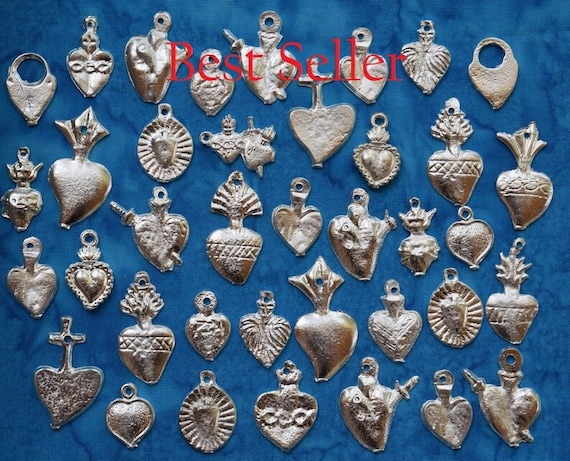The image features a blue marbled background with darker blue blotches. Scattered across the background are around 40 intricate silver pendants, each equipped with a small hole at the top, suggesting they are designed to be strung onto necklaces or bracelets. The pendants come in various shapes, predominantly heart-shaped, but some appear as spades, reminiscent of playing cards, while others resemble celestial suns or even fruits. There are pendants with crosses intersecting hearts and some adorned with chains, crosshatches, or dagger-like symbols piercing through them. Positioned at the top center of the image, bold red text declares "Best Seller," slightly overlaying the top row of pendants, indicating these items might be marketed on platforms like eBay or Etsy.